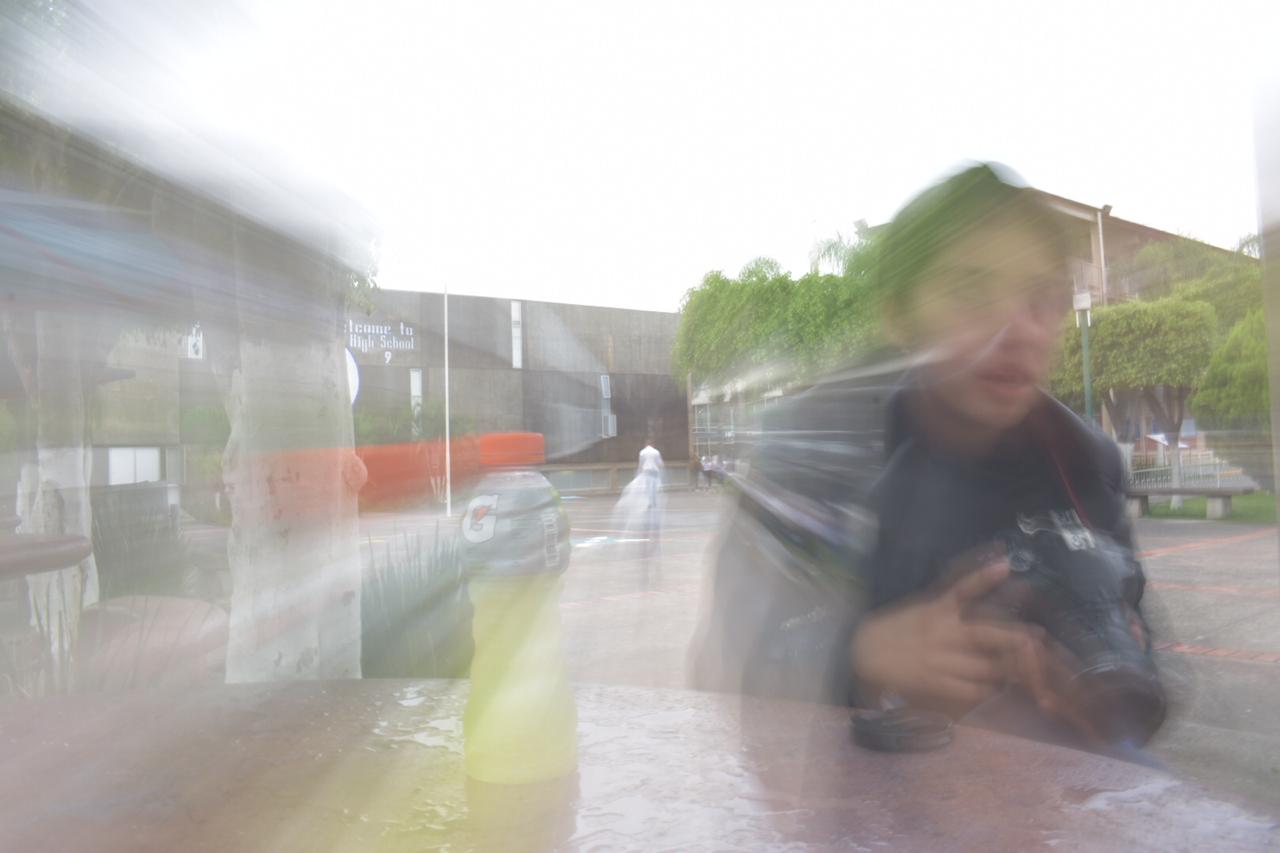In this extremely blurry and artistic daytime photograph, the primary focus appears to be on a young man seated at a rough, pinkish table in the foreground. The individual, seemingly Asian, is dressed in a black shirt with a shawl draped over his shoulders and is holding a large, high-end camera, with the lens resting on the table. Centered on the table is a yellow Gatorade bottle with an orange top. The background fades into a ghostly blur with radial lines emanating from the center, making it hard to distinguish specific details. However, some elements can be identified, such as the green hues of trees and what appears to be bushes, strawberries, and buildings. On the left and in the distance, a person dressed in white is walking away, adding to the spectral quality of the image. Despite the overwhelming blur and brightness, these focal points create an intriguing and mysterious scene.